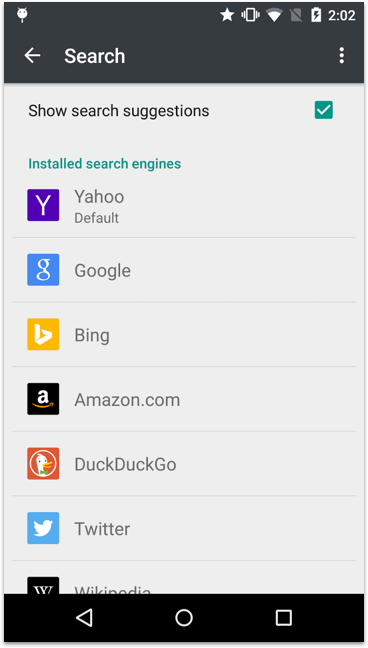A screenshot from a smartphone settings menu illustrating the search engine configuration. 
In the top horizontal black bar, roughly an inch thick, a logo is visible on the upper left corner and the time "2:02" along with battery percentage, Wi-Fi signal strength, and other icons are displayed on the upper right corner. Below this bar, a white text field labeled "Search" is present, with a left-pointing arrow next to it.

The majority of the screen is occupied by a large gray box which contains various settings. Directly below the "Search" field, a section labeled "Show search selections" is displayed in black text with a green check mark to the right. Beneath this, in bold bluish-green text, the phrase "Installed search engines" is prominent.

Further down, there are seven rows listing different search engines on the left side of the screen. The list includes:
1. Yahoo - marked as the default search engine.
2. Google.
3. Bing.
4. Amazon.com.
5. DuckDuckGo.
6. Twitter.
7. Wikipedia.